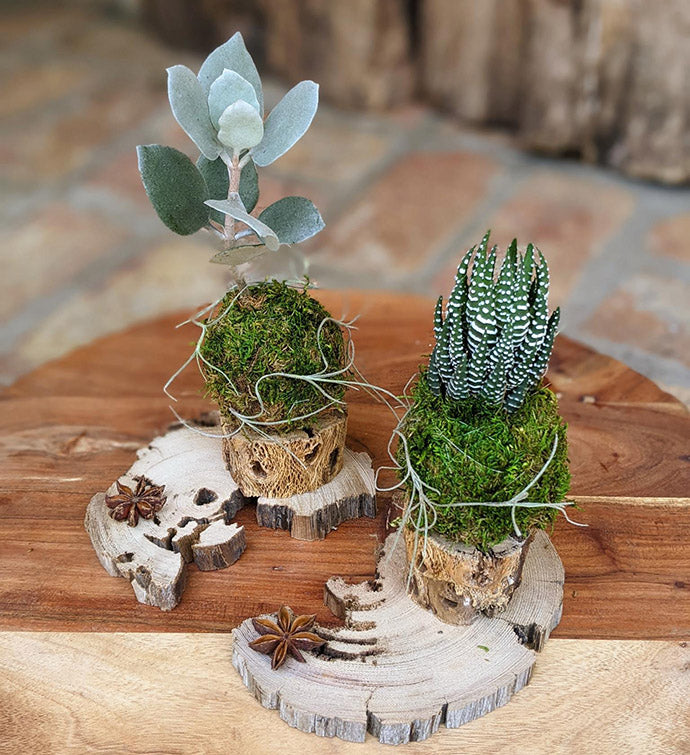The photograph captures an outdoor patio scene with natural lighting, providing a glimpse of a cozy and rustic setting. The blurred background showcases a floor made of large red bricks with gray grout, leading up to what appears to be a wooden wall or brown curtains in the upper right corner. Central to the image is a small, circular wooden table composed of horizontal planks, with the front-most plank being a light tan color and the remaining ones in a reddish-brown hue.

Dominating the table are two distinct wooden pieces that resemble split parts of a tree trunk, each adorned with a star-shaped accent at the front. These pieces are placed diagonally with a break running from the lower left to the upper right, creating two separate sections. Each trunk segment features a small round base with a pot holding a different type of plant. 

On the right side, there's a plant with green elongated leaves marked by white horizontal stripes and dots, creating an intricate pattern. The left side hosts a plant with spade-shaped leaves that are light green, softened by a thick coat of white fuzz. Both plants are positioned centrally in the image, enhancing the rustic charm of the scene with their vibrant green foliage against the earthy tones of the wood and bricks. This setting is indicative of an outdoor space meant for relaxation and quiet moments, possibly a private patio lounge.